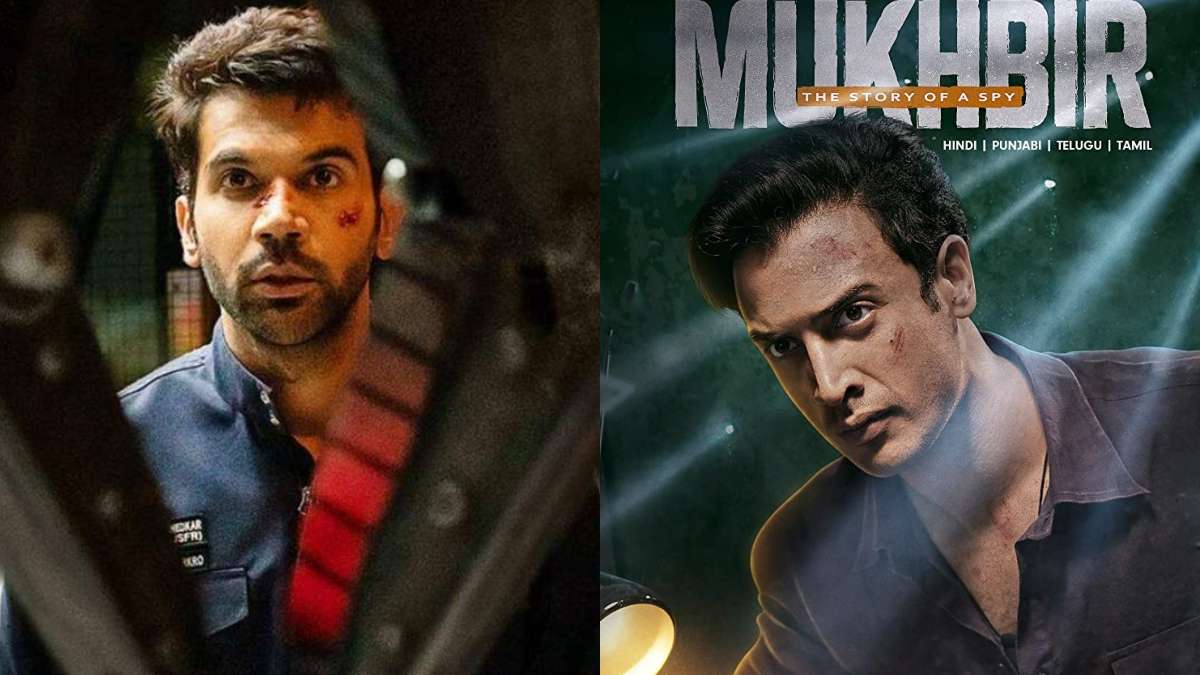The image appears to be a detailed Indian movie poster titled "MUKHBIR: The Story of a Spy." The poster is visually split into two halves. On the left side, it features a South Asian man with short, dark hair and a beard adorned with a goatee. He has visible wounds on the bridge of his nose and on his left cheek. He is wearing a dark navy uniform-like shirt with a pocket on the chest, above which there are some obscured words that suggest a name tag or job description. His image is partially obscured as if viewed through a keyhole or some type of machine.

On the right side, set against a dark green background perforated with bullet holes through which light streams, there is another South Asian man (or possibly the same man, though with a stern and more focused expression). This individual also has dark hair but lacks the stubble and facial wounds seen on the left. He is dressed in a collared shirt and is positioned looking towards the lower left corner. Large, bold letters spell out "MUKHBIR" behind his head, with a gold banner beneath that reads "The Story of a Spy." Additional smaller text below the title indicates that the film is available in multiple languages: Hindi, Punjabi, Telugu, and Tamil. The entire composition suggests an intense and gripping narrative likely centered around espionage and personal conflict.